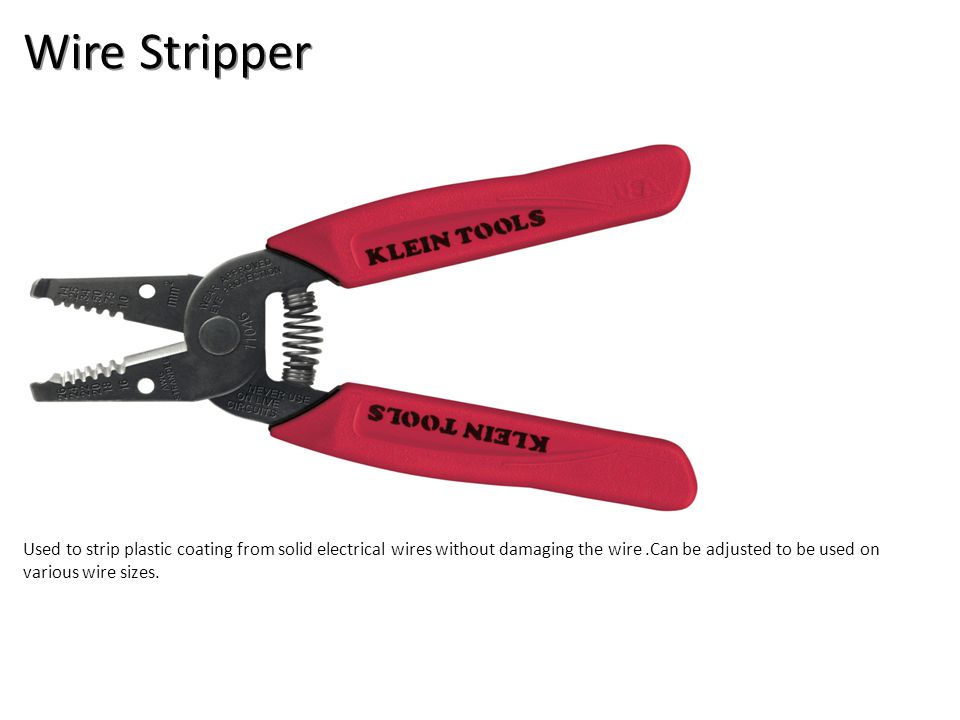This image is a detailed photograph of a wire stripper by Klein Tools, set against a white background. The wire stripper has prominent red handles, each emblazoned with the brand name "KLEIN TOOLS" in bold, black capital letters. The handles are connected to a sturdy, dark gray metal head that features lighter gray, jagged teeth designed for precise cutting. The tool includes a vertical spring that connects the two halves, facilitating smooth operation. Positioned above the wire stripper is large black text reading "Wire Stripper," with the first letter of each word capitalized. Below the tool, smaller black text explains its purpose: "Used to strip plastic coating from solid electrical wires without damaging the wire. Can be adjusted to be used on various wire sizes." The wire stripper is depicted slightly open, with its functional metal components facing left and the handles oriented to the right.